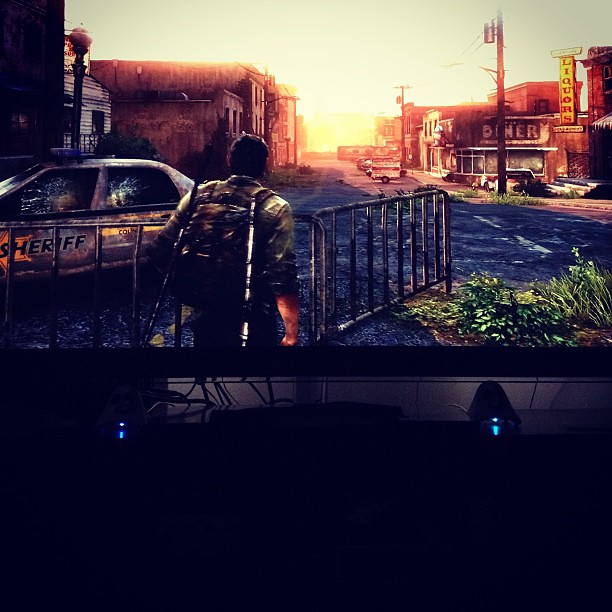In a dimly lit room that appears to be someone's bedroom or living room, a large flat-screen TV displays a scene from the video game The Last of Us. The picture seems to be a photograph taken with a smartphone, as the surrounding dark environment reveals some illuminated electrical devices, wires, and a cabinet holding various items. The game screen depicts a post-apocalyptic setting with an older man, likely Joel, wearing a backpack and walking down a deserted street. To his left is a dilapidated sheriff's car with shattered windows, and the area is surrounded by abandoned buildings, including a diner and a liquor store. The cracked pavement has overgrown greenery sprouting from it, heightening the desolate atmosphere. The darkness of the room is subtly broken by the glow of the TV, drawing focus to the immersive, realistic graphics of the game.